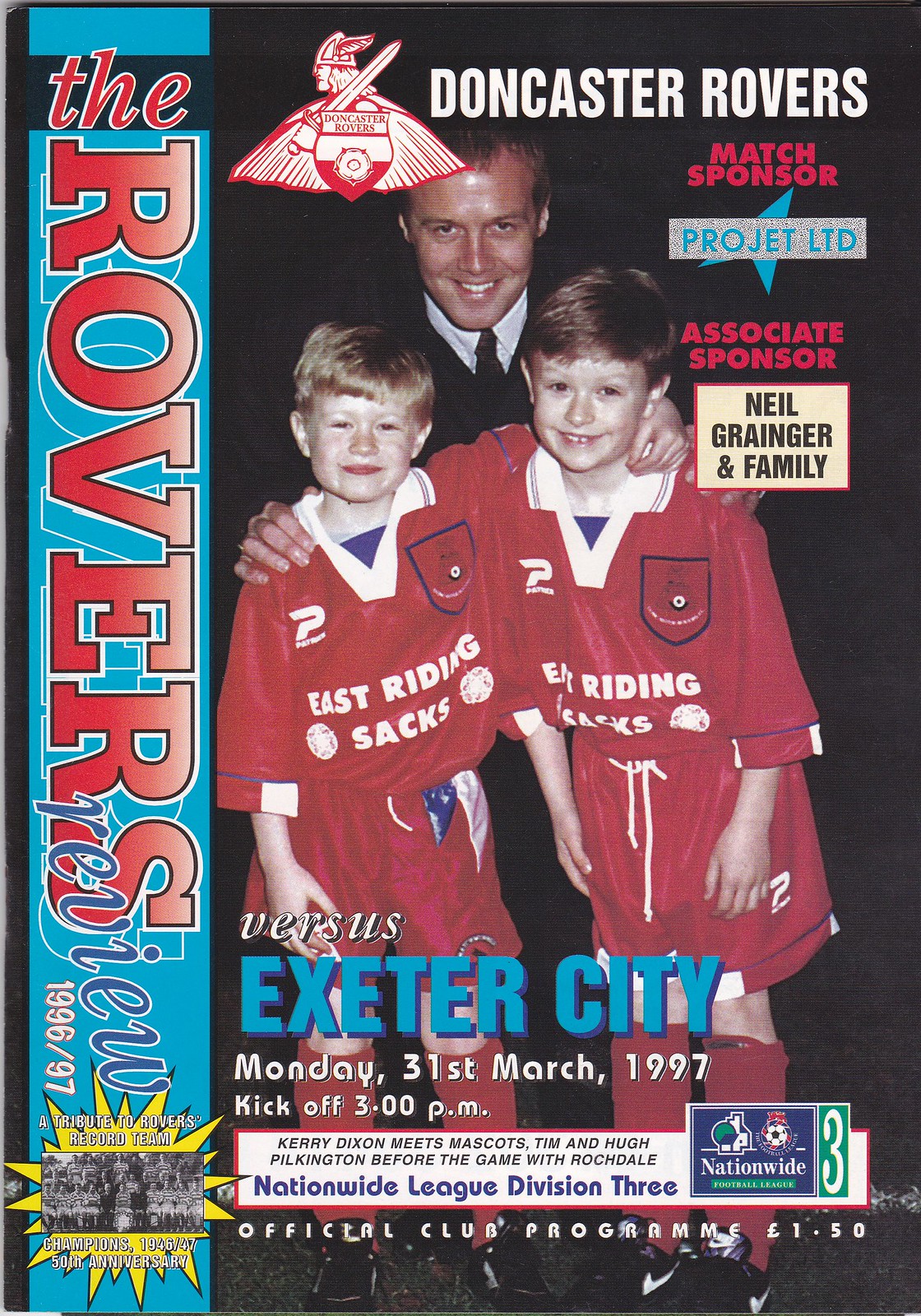The image is a portrait-oriented, official club program for the Doncaster Rovers soccer team, spanning the 1996-97 season. It features a man in a white shirt and tie, likely Neil Granger, standing behind two young boys wearing matching red soccer uniforms with "East Riding Saks" written across the front in white. The man has his hands on the boys' shoulders, and all three are facing the camera. The black background accentuates the vibrant red of the boys' uniforms and the white of the man's shirt.

On the left side, a vertical ribbon bears the text "The Rovers Review 1996-97," alongside a tribute to the Rovers' record team on their 50th anniversary. At the top of the program, the Doncaster Rovers logo is prominently displayed in red and white, with the title "Doncaster Rovers" in white text above it.

Further details include the match sponsors: Project Limited and Associate Sponsor Neil Granger and Family. Below this information, the program specifies that the game is against Exeter City on Monday, March 31, 1997, with a kickoff time of 3 p.m. Additionally, a small white rectangle at the bottom of the image mentions "Kerry Dixon meets mascots Tim and Hugh Pilkington before the game with Rochdale." The program is priced at £1.50, and a blue, white, and teal Nationwide League Division III Official Club Program logo is located in the bottom right corner.

Overall, the program paints a vivid picture of a youth soccer team event, capturing the spirit and excitement of the match day.